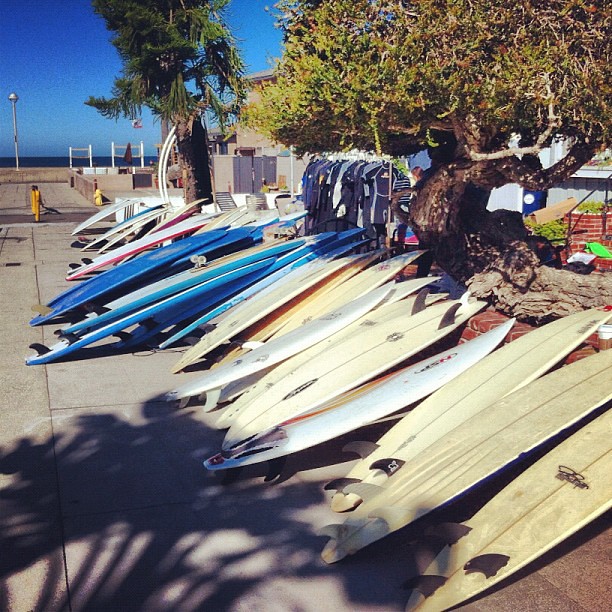The photograph captures a sunny day at the beach, where a sizable collection of surfboards, roughly between 20 to 40 in number, are neatly propped against a short brick wall. These surfboards come in a variety of colors, predominantly off-white or ivory, but also featuring blue, tan, and red-trimmed ones. They are all positioned with their fins facing up against the concrete ground. To the right of the surfboards, a large tree with a thick brown trunk and lush green leaves extends its shadow across the foreground. In the middle of the arrangement, there's a visible rack of wetsuits ready for use, hinting at the possibility that these items are available for rental or resale. The backdrop showcases a beautiful scene of electric blue skies, a vast body of water, and a blend of dark and light green trees, including a palm tree, which add to the tropical ambiance. Additionally, there's a streetlight on a concrete barrier and some outdoor furniture visible in the distance, contributing to the leisurely atmosphere of this beachside setting.